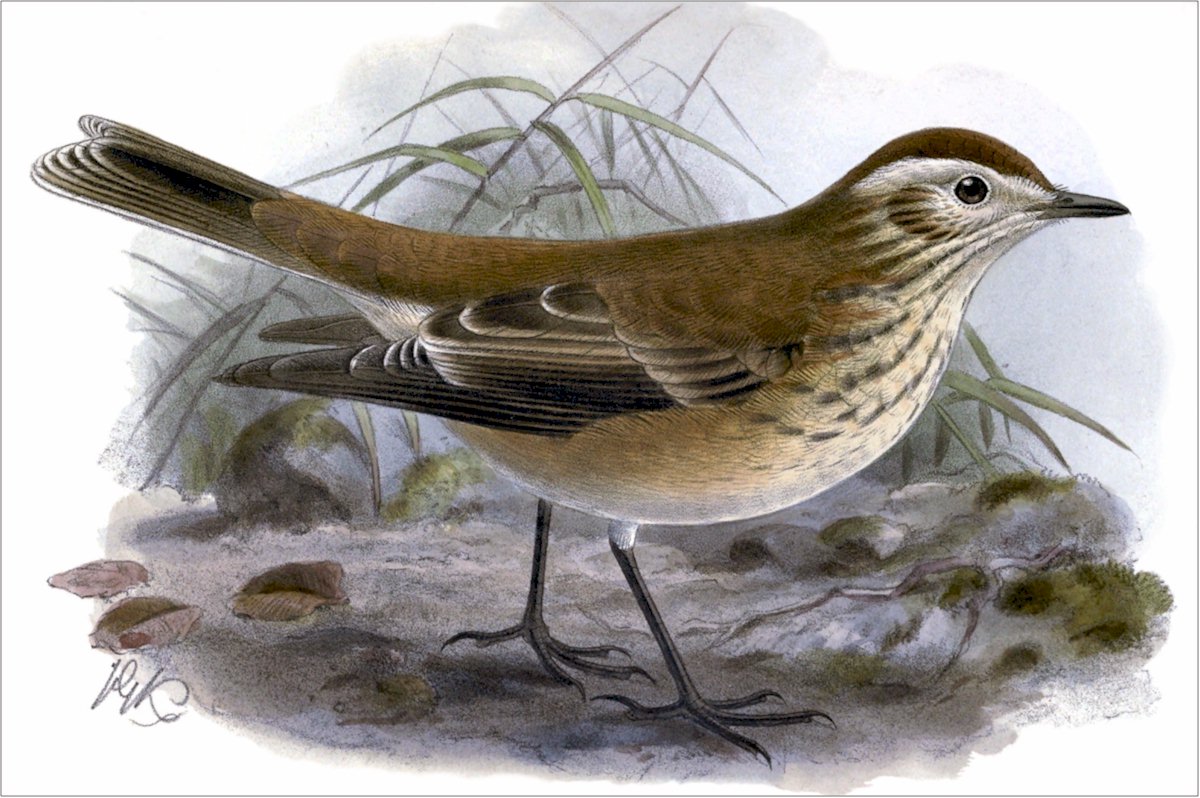This detailed, up-close painting of a brown bird showcases a striking contrast against an all-white background. The bird, which appears to be a blend of light brown and tan shades, features a white patch around its eyes, adding a touch of brightness to its otherwise earthy palette. Its beak, short and pointed, along with its eyes, are both jet black, highlighting its sharp, attentive expression. The crown of the bird’s head is brown, flowing seamlessly into the light brown and tan hues that cover its body. The wings exhibit a gradient from brown near the body to black at the tips, accented with light tan streaks, while the tail feathers show a combination of dark brown and black strap-like patterns. The bird stands confidently on the ground, surrounded by a few blades of grass and scattered brown leaves. The painting is signed by the artist, although the signature is not legible. The detailed depiction, reminiscent of wildlife illustrations in books, captures the essence of the bird's natural beauty and habitat.